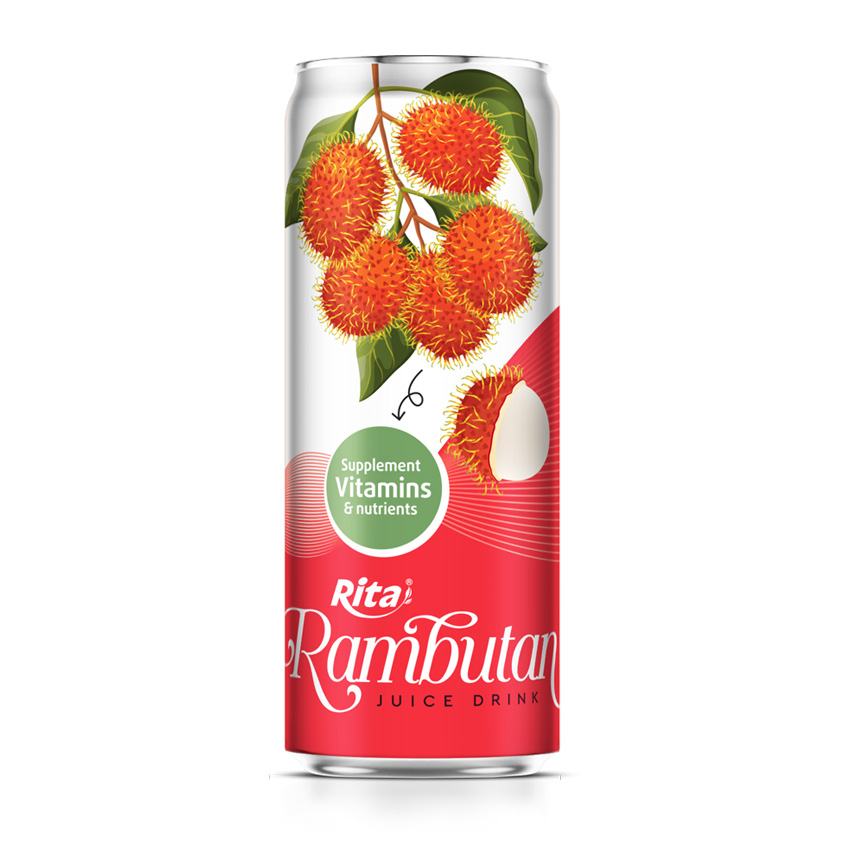The image shows a tall, cylindrical can of a juice drink. The can features a prominent illustration of rambutan fruits, which are round and orange with distinctive yellow spikes and red caps. These fruits are depicted hanging from a thin branch adorned with several green leaves. In the middle of the can, a light green circle contains white text that reads "Supplement Vitamins and Nutrients." The can transitions from white at the top to red at the bottom. At the bottom, the brand name "Rita" and the product name "Rambutan" are displayed in white text, with "Rambutan" written in an italicized, serif font. Below this, "Juice Drink" is printed in black, all-caps, sans serif font.